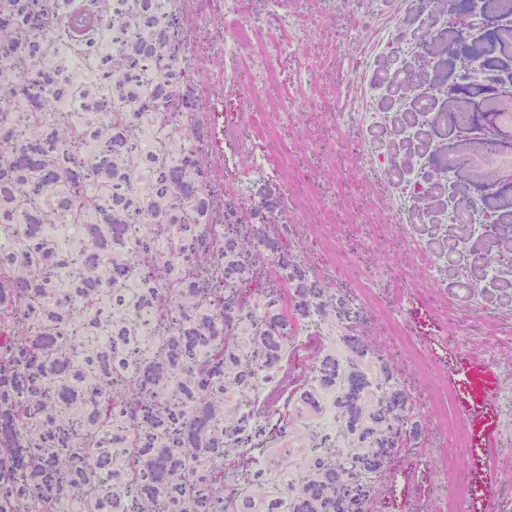This image appears to be a highly detailed microscopic slide, potentially of a blood vessel or cellular structure. Dominated by a vibrant palette of pinks, lavenders, and whites, the photograph is square and free of any explanatory text. From the lower right corner, a bright pink, river-like structure flows upward, terminating near the middle of the upper part, slightly to the right. This pink strand is intricately interwoven with off-white lines and occasional darker pink specks. Surrounding this central feature, the image is speckled with clusters of small purple and lavender cells, creating a textured pattern that extends from the top left down to the middle lower center of the image. The far top right is marked by larger, almost blob-like patches in similar hues, lending the composition an artistic yet scientific aesthetic.